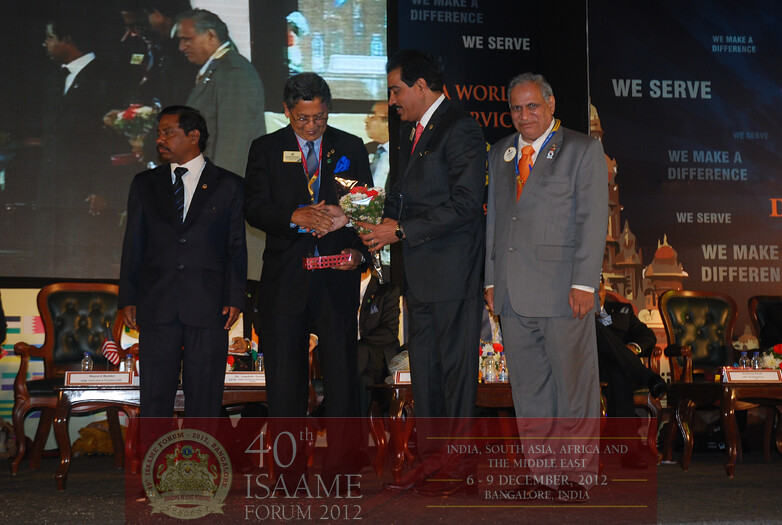This horizontal snapshot captures four distinguished gentlemen in suits, standing on a stage in Bangalore, India, at the 40th ISAAME Forum 2012, held from December 6-9. In the background, a large screen projects the men for the audience's better view, alongside banners and intricate red text detailing the event. From left to right, the first gentleman is of dark skin tone with a black suit, striped black tie, white shirt, dark hair, and a mustache; he is looking to the left. The second gentleman, slightly older with glasses and short black hair, glances downwards while shaking hands with the third man. He wears a black suit with a blue shirt and tie, a gold name tag, and holds a blue handkerchief protruding from his pocket. The third gentleman, taller than the second, sports a red tie, white shirt, dark suit, and a bouquet of flowers in his left hand, complemented by his short black hair and mustache. Finally, the man on the far right, who appears the oldest with gray hair, dark eyebrows, and wearing a gray suit, orange tie, and white shirt, faces the camera with an unreadable expression. Behind them are wooden chairs with leather seating, adding a formal ambiance to the setting. The emblematic red banner below them reads: "40th ISAAME Forum 2012," followed by “India, South Asia, Africa, and the Middle East, 6-9 December 2012, Bangalore, India.”